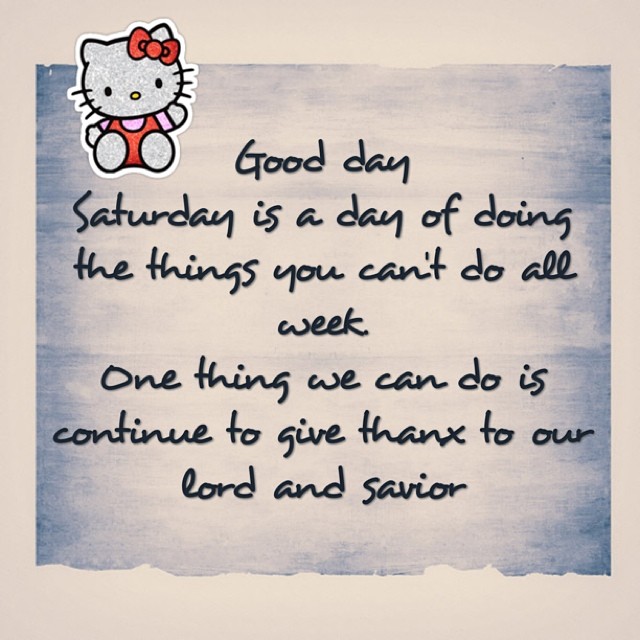The image features a piece of paper that appears to have a blue, crumpled texture. It is attached to a white, bordered background using a Hello Kitty sticker in the upper left corner. Hello Kitty, adorned with her signature red bow, red jumpsuit, and waving, accents the image charmingly. The text on the paper is handwritten in a mix of cursive and print, reading: "Good day. Saturday is a day of doing the things you can't do all week. One thing we can do is continue to give thanks to our Lord and Savior." Despite the inspirational tone, certain words like 'Good', 'Saturday', and 'One' are capitalized, while 'Lord' and 'Savior' are not. The background of the image is light gray, adding a soft contrast to the overall design.